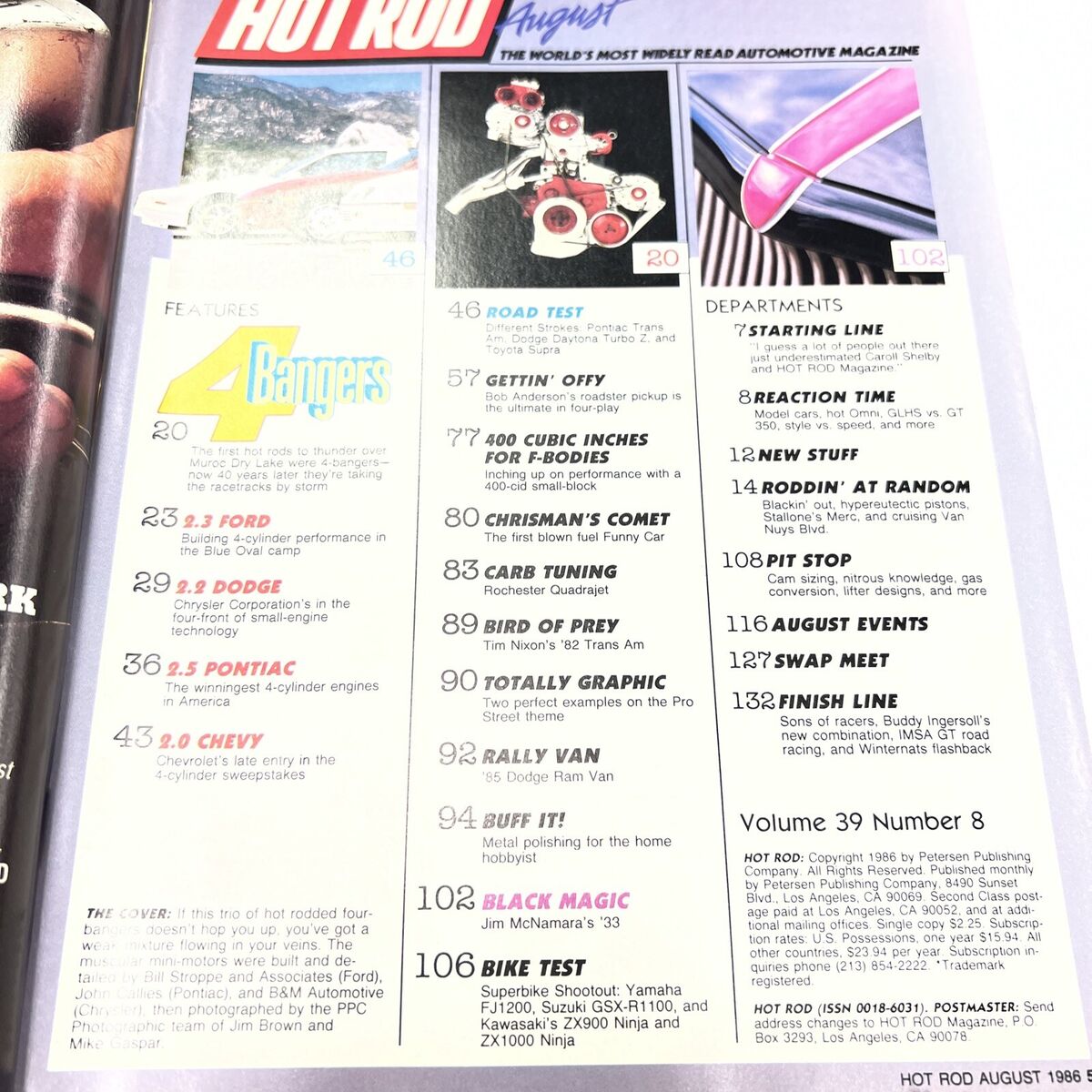Here we have an image of an open magazine featuring Hot Rod, the world's most widely read automotive magazine, specifically the August 1986 edition (Volume 39, Number 8). The cover is predominantly white with the Hot Rod logo in bold red and white at the top. The content on the page lists various articles, such as "Four Bangers," "400 Cubic Inches for F-Bodies," "Christman's Comet," "Carb Tuning," "Bird of Prey," "Totally Graphic," and more. This issue includes sections divided into three equally sized columns, each listing different features and articles with associated page numbers ranging from 20 to 132. The page captures a glimpse into a richly detailed automotive enthusiast's world, showcasing the diverse topics covered in this vintage publication.